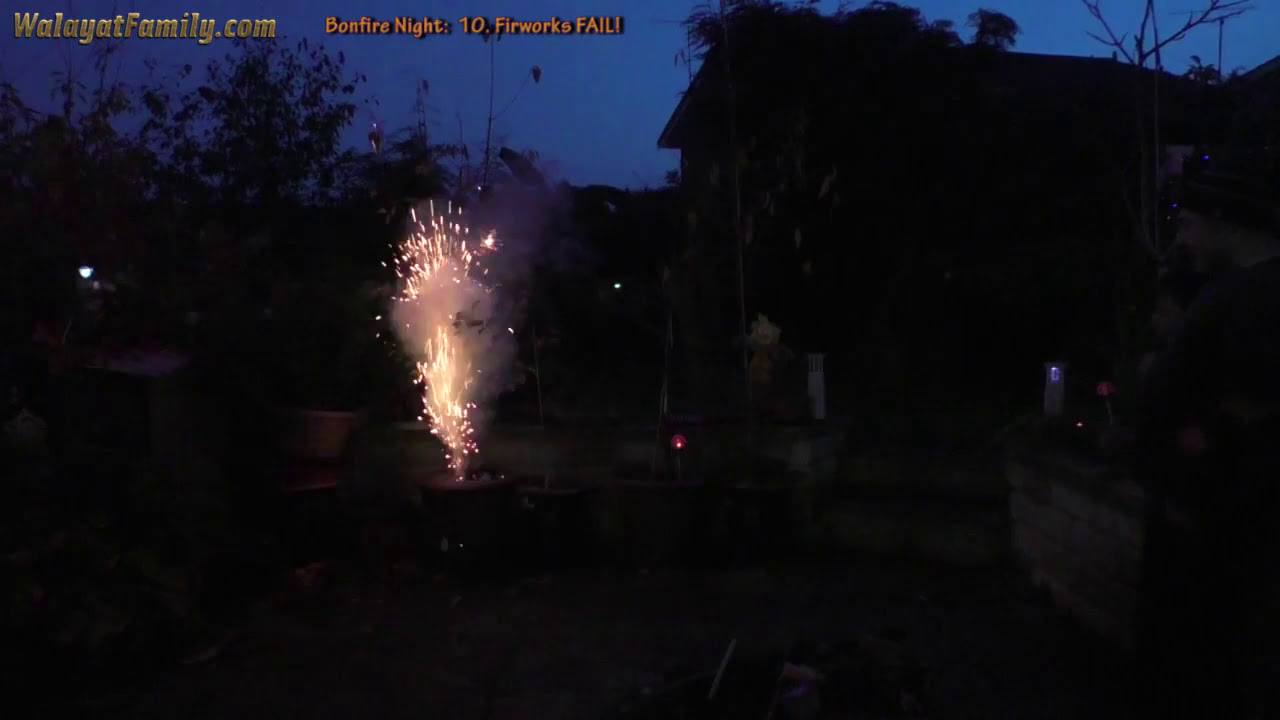The photograph captures a night-time scene dominated by the vibrant, golden sparks of an ignited firework positioned slightly left of the center. The dark blue sky serves as a contrasting backdrop. On the top left corner, text in gold letters reads "WalayatFamily.com" followed by "Bonfire Night: 10 Fireworks Fail!" Below the fireworks, the dim silhouettes of houses and trees can be faintly seen, with two steps discernible to the right of the sparkling display. The image is cloaked in darkness, making the firework and the golden text the most distinct elements, while the rest of the scene remains shadowy and indistinct.